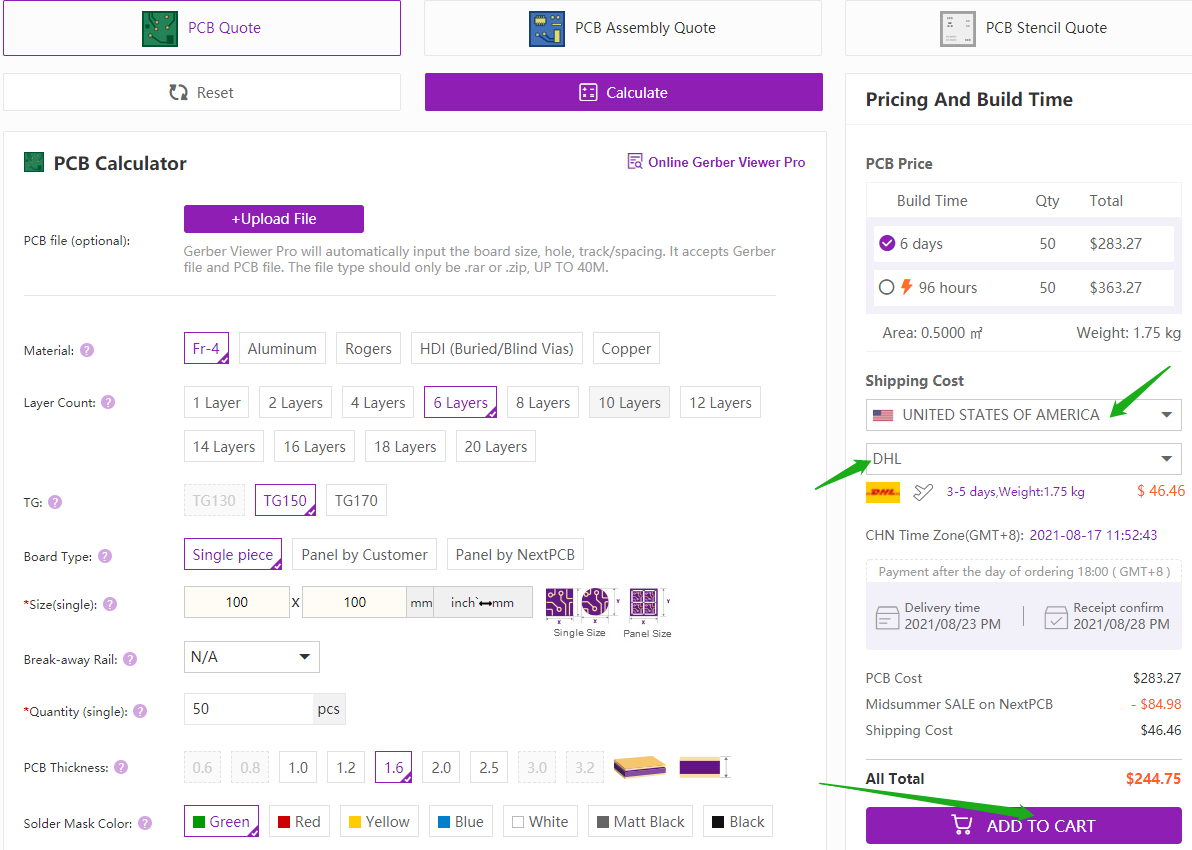This image depicts a screenshot of a program or web page dedicated to PCB (Printed Circuit Board) services, showcasing three main tabs across the top: "PCB Quote," "PCB Assembly Quote," and "PCB Stencil Quote." Below these tabs, there are reset and calculate buttons, with the calculate button currently highlighted in purple, indicating it has been selected. 

The screenshot's right-hand side features a column titled "Pricing and Build Time," providing detailed cost information including PCB Price, Shipping Cost, and an itemized total price of $244.75. There is also a prominent "Add to Cart" button located within this section.

Dominating the left-hand side is a section titled "PCB Calculator," listing various options and statistics related to the PCB order. These options, arranged in a vertical menu from top to bottom, include: PCB File, Material, Layer Count, TG (Glass Transition Temperature), Board Type, Size, Breakaway Rail, Quantity, PCB Thickness, and Solder Mask Color. Each of these selectable options allows users to specify the various parameters of their PCB order.